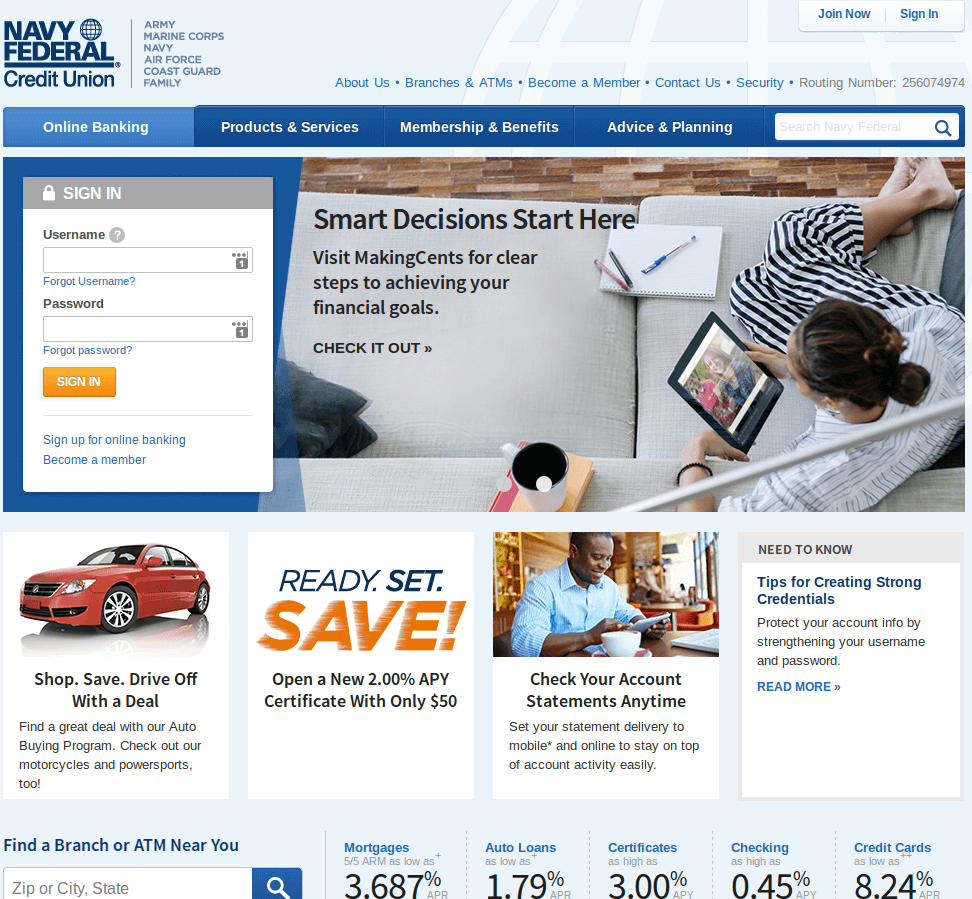**Navy Federal Credit Union Website Overview**

In the upper left-hand corner of the Navy Federal Credit Union website, there is a distinct round logo featuring a white circle at its center. The navigation menu lists options for different branches of the U.S. military, including Army, Marine Corps, Navy, Air Force, Coast Guard, and a category labeled "Family." 

A sub-menu includes links for "About Us," "Branches and ATMs," "Become A Member," "Contact," and "Security." Additionally, a routing number is displayed in gray in this section. In the upper right-hand corner, there are options to "Join" and "Sign In."

The website features various sections such as "Online Banking," "Products and Services," "Membership and Benefits," and "Advice and Planning." There is also a search bar available for user convenience.

A prominent white pop-up box with a gray header is present on the screen, titled "Sign In." It contains a lock icon and prompts users to enter their username and password. An orange "Sign In" button is available for submission.

The upper portion of the website showcases an overhead image of a woman sitting on a light gray couch. She is wearing black and white striped pants and a white shirt with black lines. Her black hair is tied in a ponytail as she looks at an iPad displaying an image of a white man and woman. She is holding a white coffee cup that rests on a book.

Below this image, there are advertisements, including one featuring a red car with the slogan "Ready, Set, Save." Another ad promotes checking account statements at any time. Additional content offers tips on creating strong credentials and information on locating branches by entering a city and state.

At the bottom of the page, current rates for mortgages, auto loans, certificates, checking accounts, and credit cards are displayed.